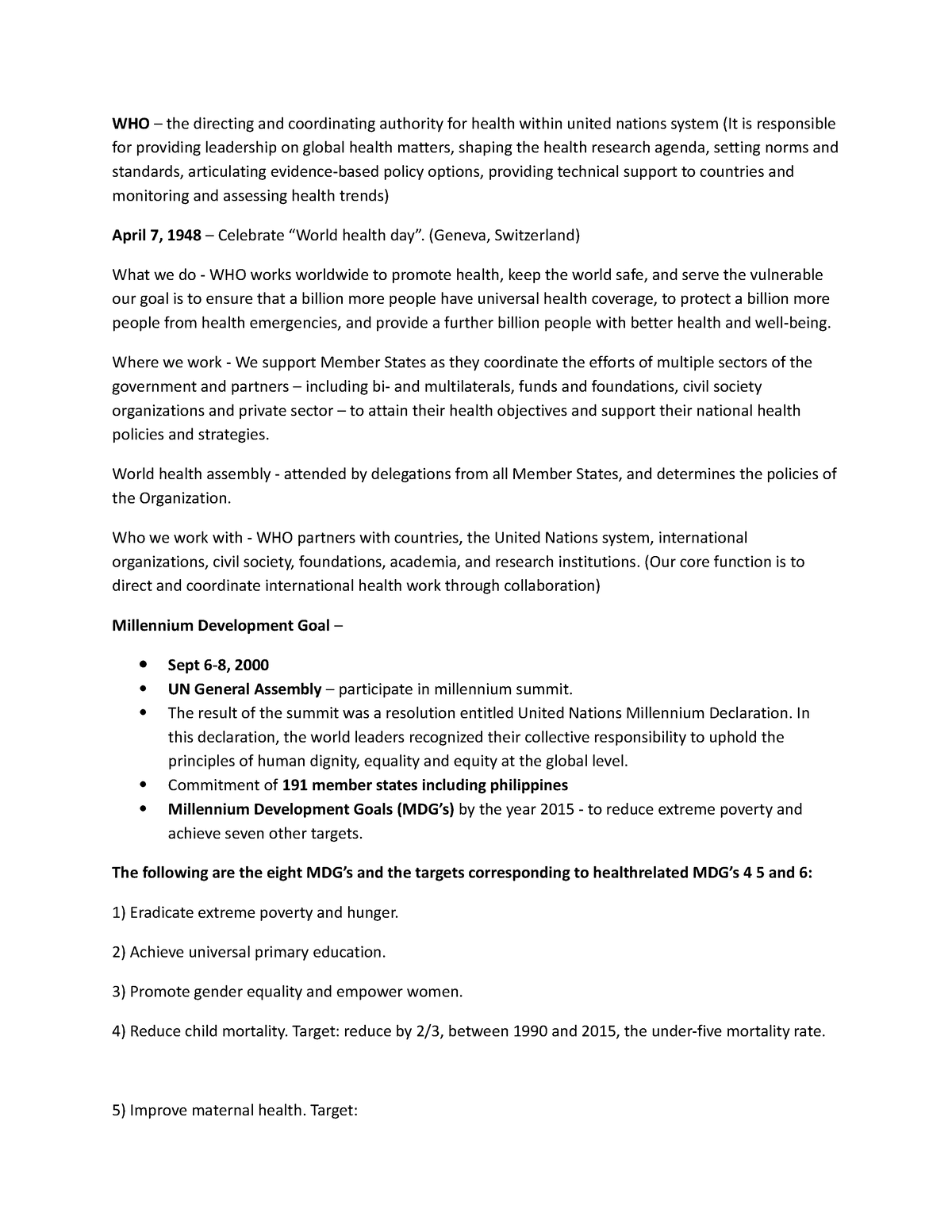The image contains black text on a white background with no border. In the upper left corner, "WHO" is prominently displayed in bold letters, representing the World Health Organization, the directing and coordinating authority for health within the United Nations system. The text further introduces the organization and its role.

The subsequent paragraph highlights a significant date: April 7th, 1948, marking World Health Day in Geneva, Switzerland, which is recognized as the founding date of WHO.

Following this, the text provides an overview of WHO and its mission. Further down, it references the Millennium Development Goals (MDGs), specifically mentioning a key event: the UN General Assembly from September 6th to 8th, 2000.

The image then lists the eight MDGs and emphasizes the health-related targets of MDGs 4, 5, and 6. The enumerated goals are:

1. Eradicate extreme poverty and hunger.
2. Achieve universal primary education.
3. Promote gender equality and empower women.
4. Reduce child mortality, with a target to reduce the under-five mortality rate by two-thirds between 1990 and 2015.
5. Improve maternal health.

In summary, the image provides detailed information about the World Health Organization, its founding, the Millennium Development Goals, and specific health-related objectives.